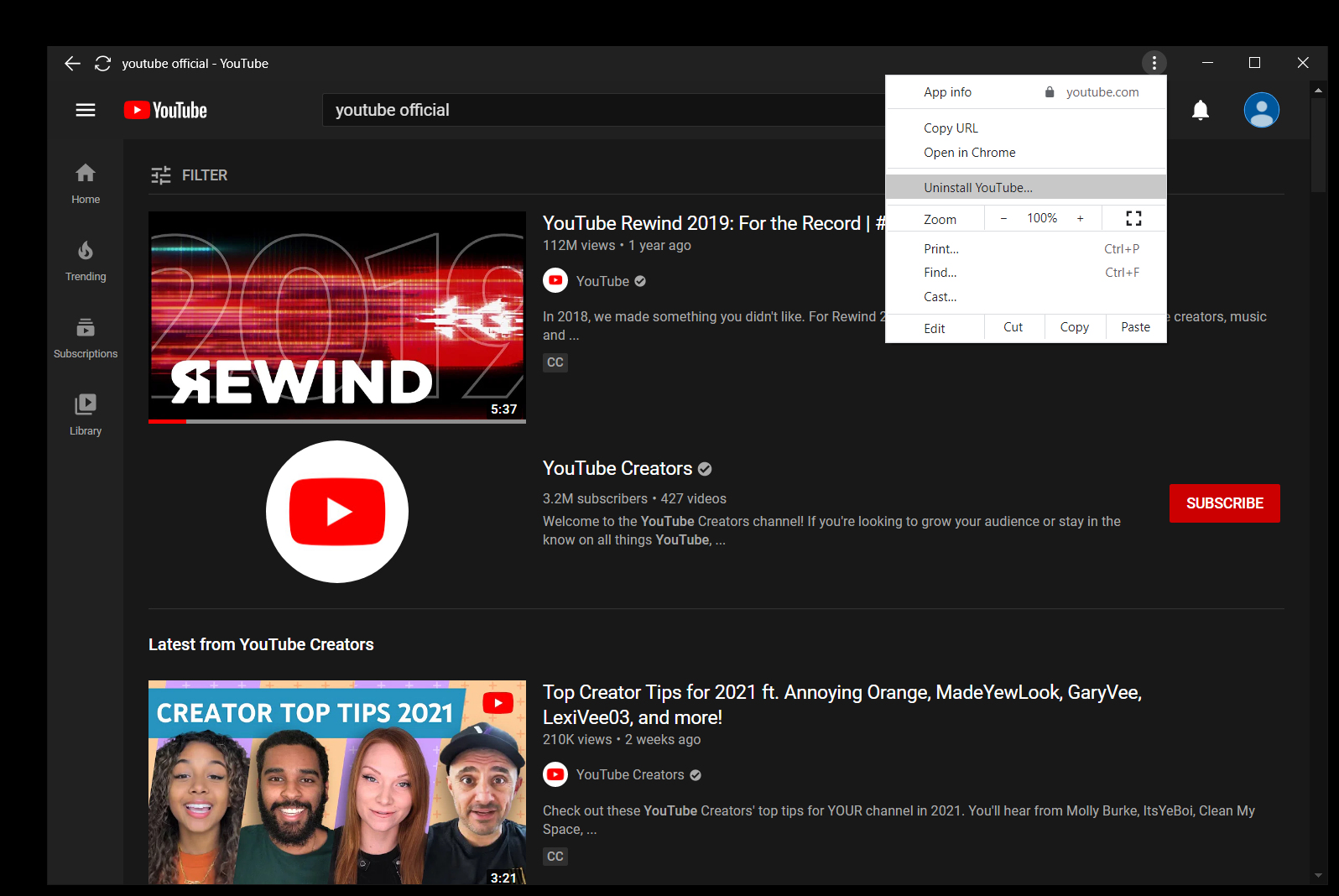The image features a black background with various YouTube-related elements prominently displayed. On the left side, there's a red box containing a small white play arrow icon, representing YouTube. To the right of this icon, the word "YouTube" is displayed in white text. Further to the right, there's a black search bar with the text "YouTube official" inside it. Adjacent to the search bar is a white box labeled "App info," and highlighted in gray is the option "Uninstall YouTube."

In the center of the image, a red box with white text reads "2012 rewind," with the "R" character facing backward. Below this box, the video synopsis states "YouTube Rewind 2019," with additional metadata indicating "112M views" and "1 year ago."

Below the synopsis, there's a white circle containing a red square with a small white play arrow inside it. To the right of this circle, the text "YouTube Creators" appears in white, along with further details indicating "3.2M subscribers" and "427 videos." To the far right, there is a red box with the option to "Subscribe."

At the bottom of the image, a video thumbnail features four different people with the title "Creator Top Tips 2021." The video's duration, "3:21," is displayed in the bottom right corner of the thumbnail.